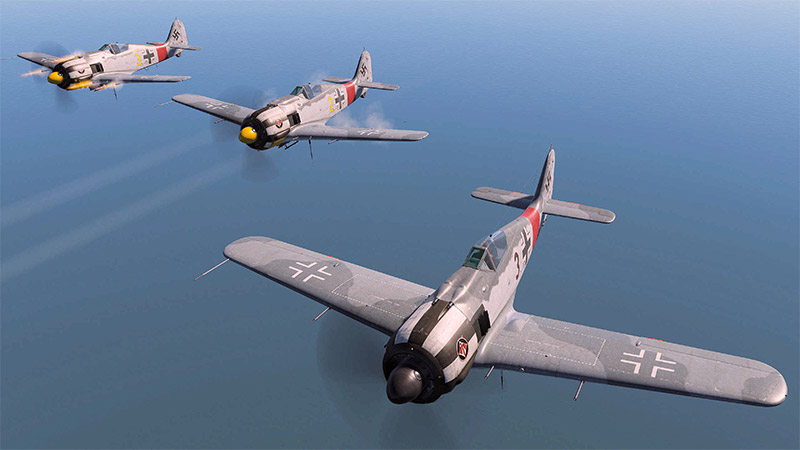This image captures three World War II German fighter planes flying in tight formation, with the photograph taken from above and to the right, providing a clear, detailed view of the planes against a bright blue background that resembles water. The leading aircraft, positioned closest and to the right, showcases a gray nose cone with black and white stripes and appears with the most detail. The two trailing planes, situated to the left and slightly back, feature yellow nose cones. Each aircraft is adorned with gray camouflage and bears an emblematic cross on the wings and tail. Distinctively, all three planes have red stripes near the tail section. The angular perspective offers a comprehensive view of the planes' upper and side profiles, showcasing their sleek design and the absence of pilots, enhancing the historical gravitas of this striking aerial image.